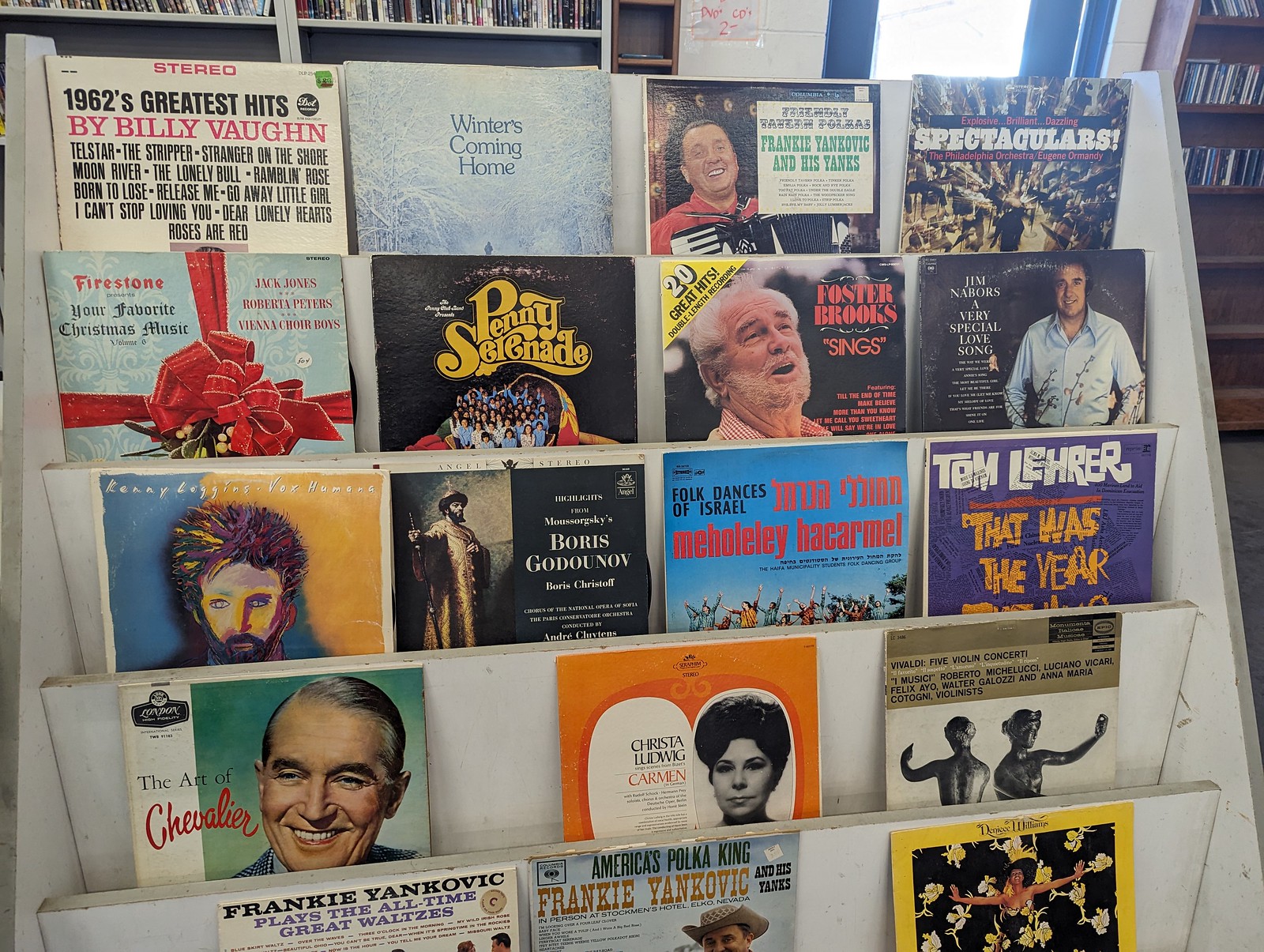The image depicts a white wooden rack, aged and slightly stained, which serves as a display for vintage record albums from the 1960s. The stand is organized into five rows, with the top three rows each holding four album covers, and the bottom two rows holding three album covers each. The album covers on display are vividly colorful, featuring a palette of blue, orange, yellow, and red. Some covers show male figures and all contain various texts and titles. Notable albums include "1962's Greatest Hits" by Billy Bond, "Winter's Coming Home" by Frankie Yankovic and his Yanks, "Spectacular" by the Philadelphia Orchestra conducted by Eugene Ormandy, "Your Favorite Christmas Music" by Firestone, "Penny Serenade," "Foster Brooks Sings," "A Very Special Love Song" by Jim Nabors, "Vox Humana" by Kenny Loggins, "Boris Gudunov" by Boris Kristoff, "Folk Dances of Israel," and "That Was the Year" by Tom Lerner. The background reveals more wooden, brown bookcases and a door with a large, bright window that adds light to the scene.